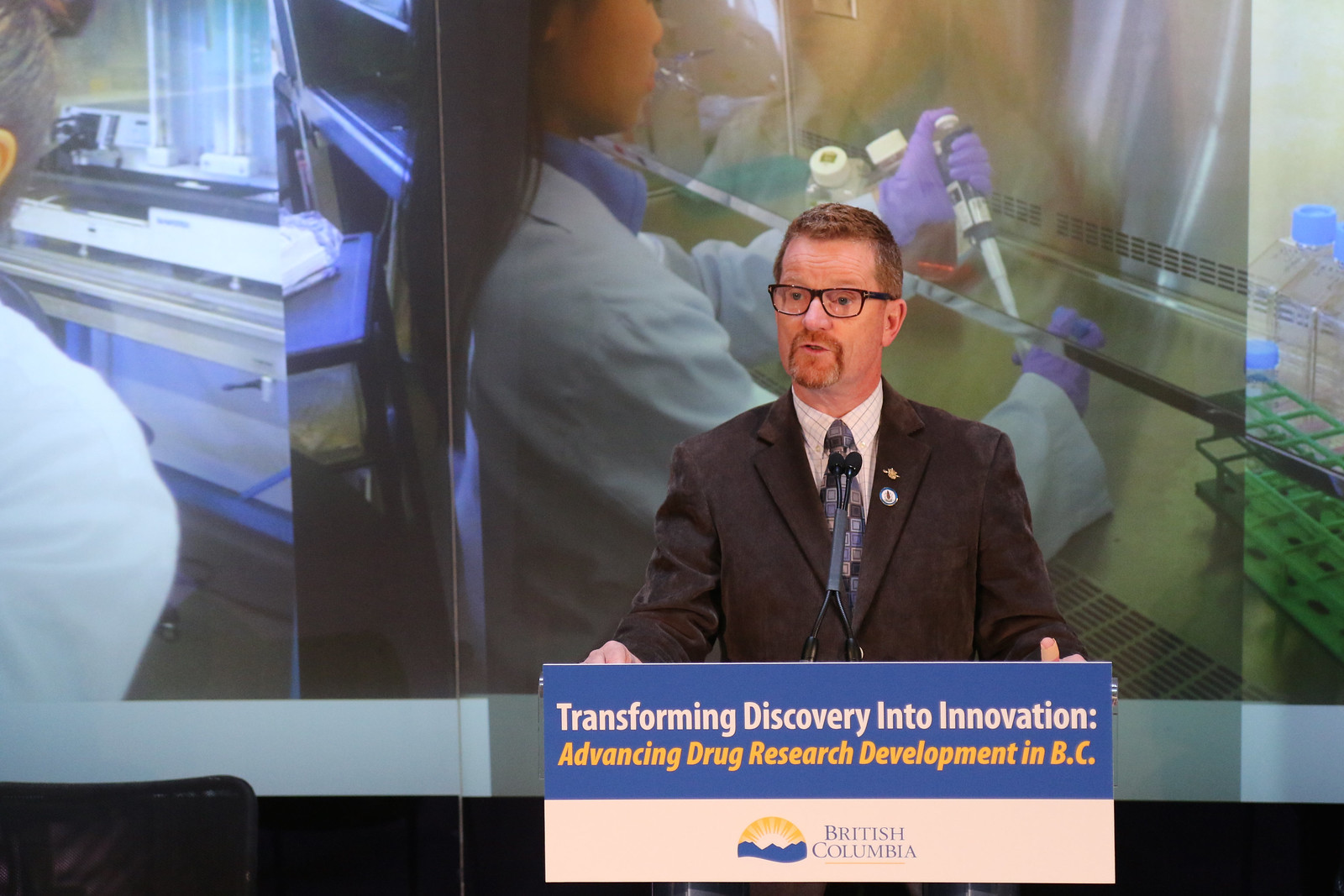This photograph captures a man in his late 40s standing at a podium, delivering a speech. He is dressed formally in a brown suit, brown tie, and an off-white shirt with brown stripes. The man has short brown hair, brown plastic glasses, and a goatee with some white around the chin area. The podium he stands behind has a prominently displayed sign that reads, "Transforming Discovery into Innovation, Advancing Drug Research Development in BC." Below this, there is a logo featuring a yellow rainbow arching over a mountain range, representing British Columbia.

The background features a projection screen with images of lab technicians engrossed in their work. One technician is adding fluids into test tubes while another peers intently through a microscope. Other details include a woman in a lab coat handling a syringe, with test tubes and containers arranged meticulously around her, suggesting a highly controlled and precise environment.

The scene likely represents a convention or formal event focused on drug research and development, highlighting advanced scientific efforts in British Columbia. The speaker's serious demeanor and the detailed imagery of laboratory activities underscore the significance of the topic being addressed.